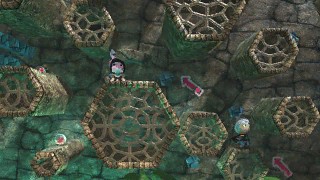Here's a detailed caption for the image:

"A side-view screenshot of a video game featuring a character scaling intricate block towers. The towers, constructed from brown latticework, create a visually appealing pattern. Clad in a pink and black outfit with a matching hat and a distinctive tail, the character climbs the structure, navigating ledges adorned with hearts encased in bubbles. Red arrows guide the player upward, indicating the path to follow. The background showcases a stone wall overgrown with patches of lush green moss, adding a touch of natural beauty to the scene."